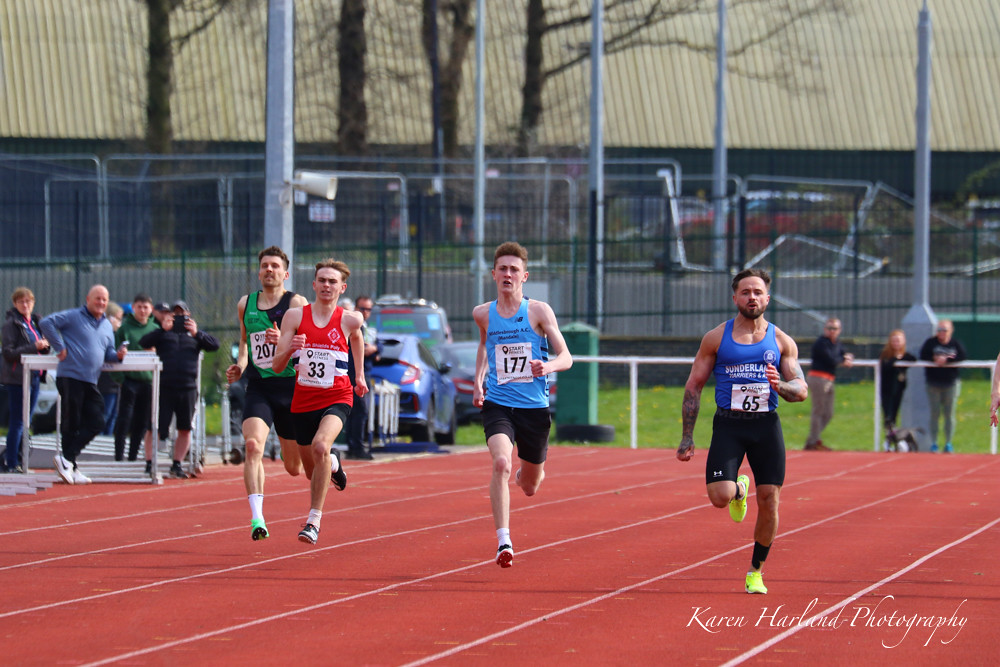This dynamic photograph captures a long-distance footrace in progress on a well-maintained burnt orange track with white stripes. The race features four male runners, all of whom are airborne except for the leading runner, whose left foot touches the ground. The participant in the lead, wearing black shorts and a dark blue tank top numbered 65, is an African-American man with black hair, a mustache, and a beard, exuding muscular athleticism. Running behind him are three Caucasian men: directly to his left is a runner in black shorts and a light blue tank top with the number 177, apparently in second place; to his further left is a runner in black shorts and a red tank top with the number 33; and furthest to the left, seemingly in fourth, is a runner wearing black shorts and a black and green tank top with the number 207.

Spectators, including what appears to be a coach holding a stopwatch, line the track. The background features a green grass field bordered by a wrought iron fence, behind which stands a two-story building with a beige-colored slat roof. Further beyond, the scene includes several large trees and a few scattered poles, as well as what might be temporary fencing or a seating area. The bottom right corner of the photograph bears the signature "Karen Harland Photography" in cursive script.